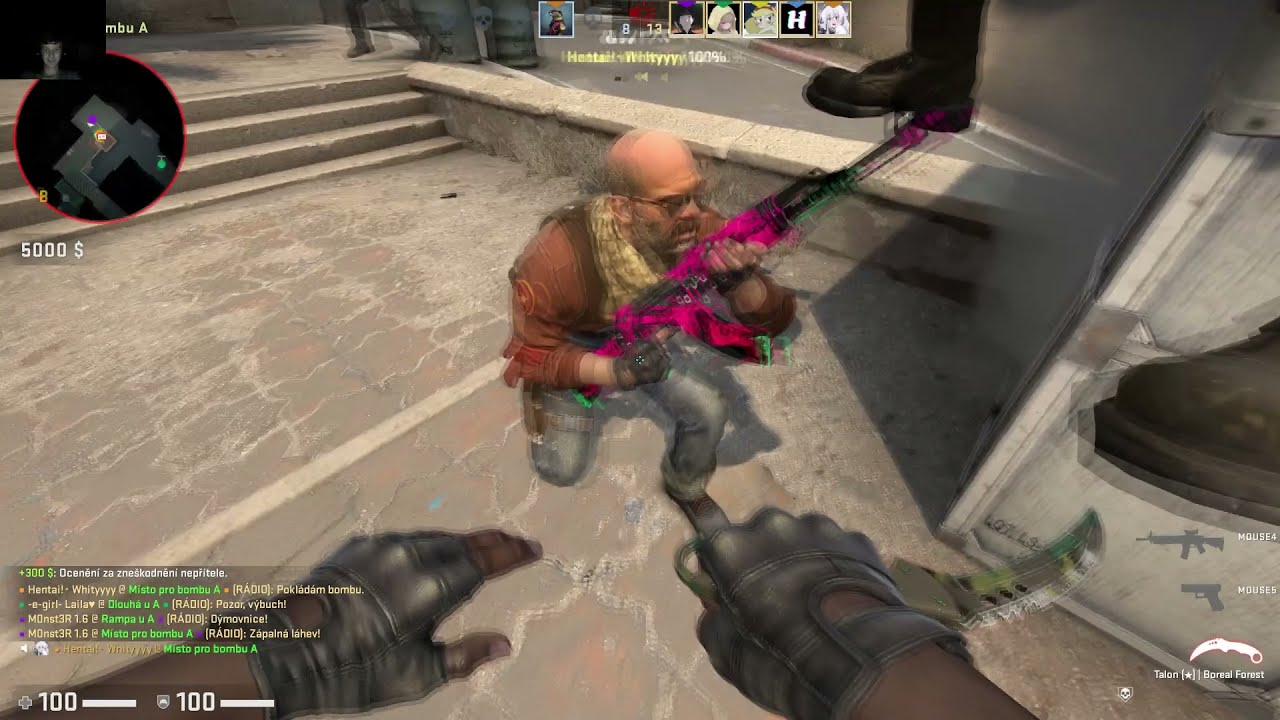The image is a detailed screenshot from a first-person shooter video game bearing a resemblance to Counter-Strike. It features a central character, a bald man with wisps of gray hair and light skin, wearing sunglasses, a brown jacket, blue-gray pants, and black shoes. He sports a white scarf around his neck and black gloves. The character is kneeling on one knee, looking upward with a hot pink assault rifle, similar to an AR-16 or AK-47, aimed ahead. The setting appears to be a dingy, dungeon-like hall with sandy brick walls crisscrossed by cracks. 

In the lower part of the image, two hands extend into the frame, covered in black, fingerless gloves and with the right hand holding a knife. In the top-right corner, a picture likely showing the player appears, along with an icon of what seems to be a desk item. To the right, there's a white cabinet or refrigerator adorned with gun images. Additional game interface elements include a mini-map in the top-left corner and a kill feed or chat in the bottom-left. The right side also displays various icons for guns and a knife similar to the one in the player's first-person perspective.